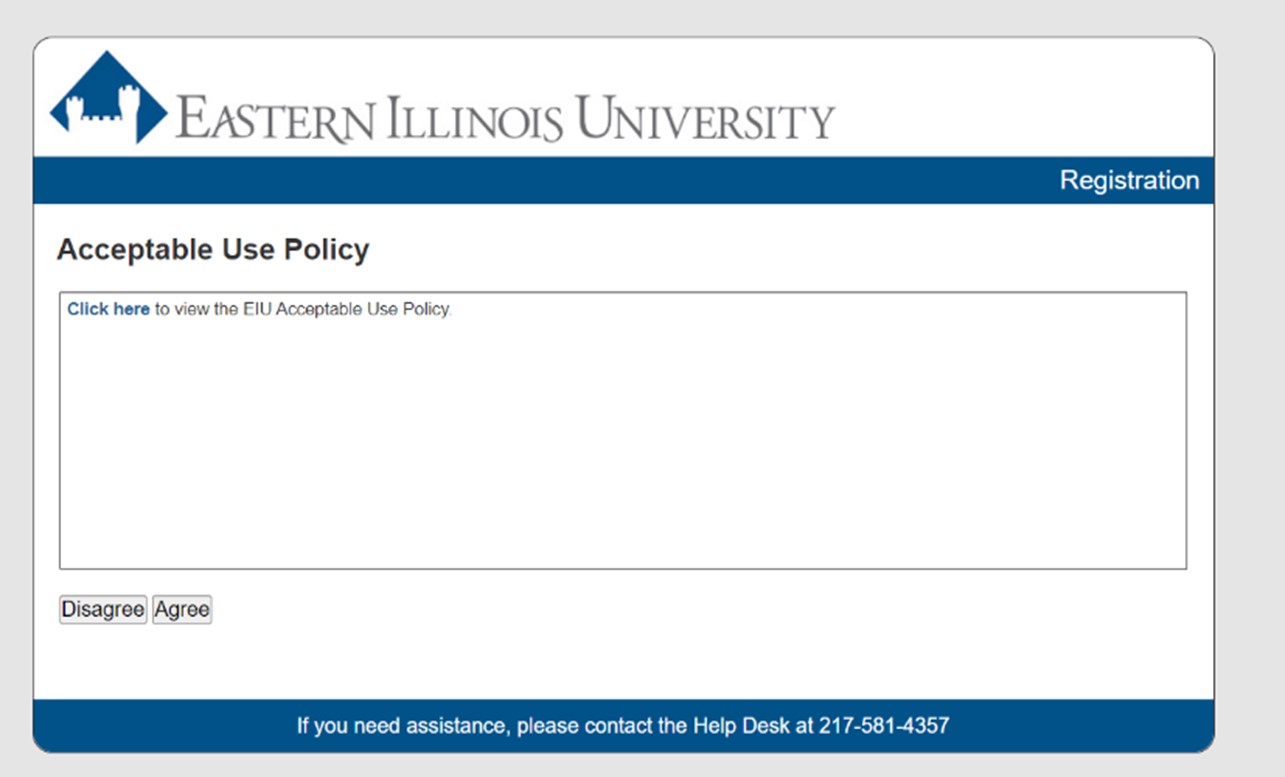This image is a cropped screenshot of the registration page from the University of Eastern Illinois' website. Prominently displayed in the top left corner is the Eastern Illinois University logo, followed by the institution's name in large, striking blue letters. Directly beneath this header, a blue horizontal bar extends across the page from left to right. On the right side of this bar, the word "Registration" is prominently displayed in bold white letters.

The section below features a white background. At the top left of this area, "Acceptable Use Policy" is written in bold black letters. Centrally located on this white background is an expansive text box. At the top of this box, there is an instruction in bold blue font that reads "click here to view the EIU Acceptable Use Policy," while the rest of the box remains empty.

Towards the bottom left of the text box are two buttons: the gray "Disagree" button and, to its right, the "Agree" button. Below these buttons, another blue horizontal bar is located at the bottom of the box. Centered on this bar is a message for assistance: "If you need assistance please contact the help desk" followed by a contact phone number.